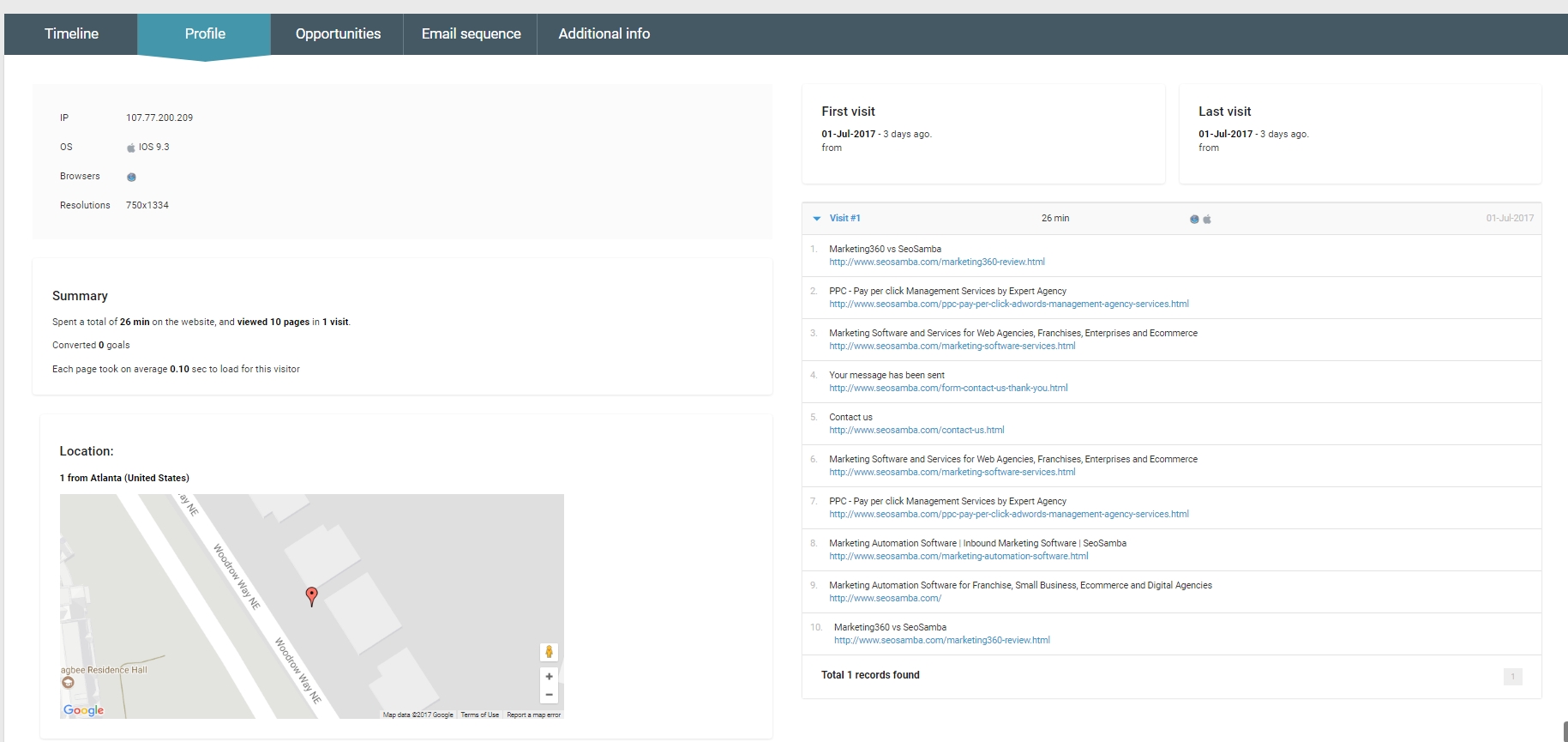The screenshot showcases a webpage interface featuring a dark gray navigation bar at the top, containing five buttons with white text: "Timeline," "Profile," "Opportunities," "Email Sequence," and "Additional Info." The "Profile" button is currently selected. 

In the bottom left corner of the screen, there's a map with a single pinpoint, labeled with the text "Location" above it and additional smaller text providing more details about the pinpointed location. Above this map section, there is a "Summary" section with three lines of descriptive text.

On the right side of the page, there is a "First Visit" field displaying a date, followed by a "Last Visit" field with another date. Below these fields, there are multiple drop-down boxes catering to additional data and options for user interaction.